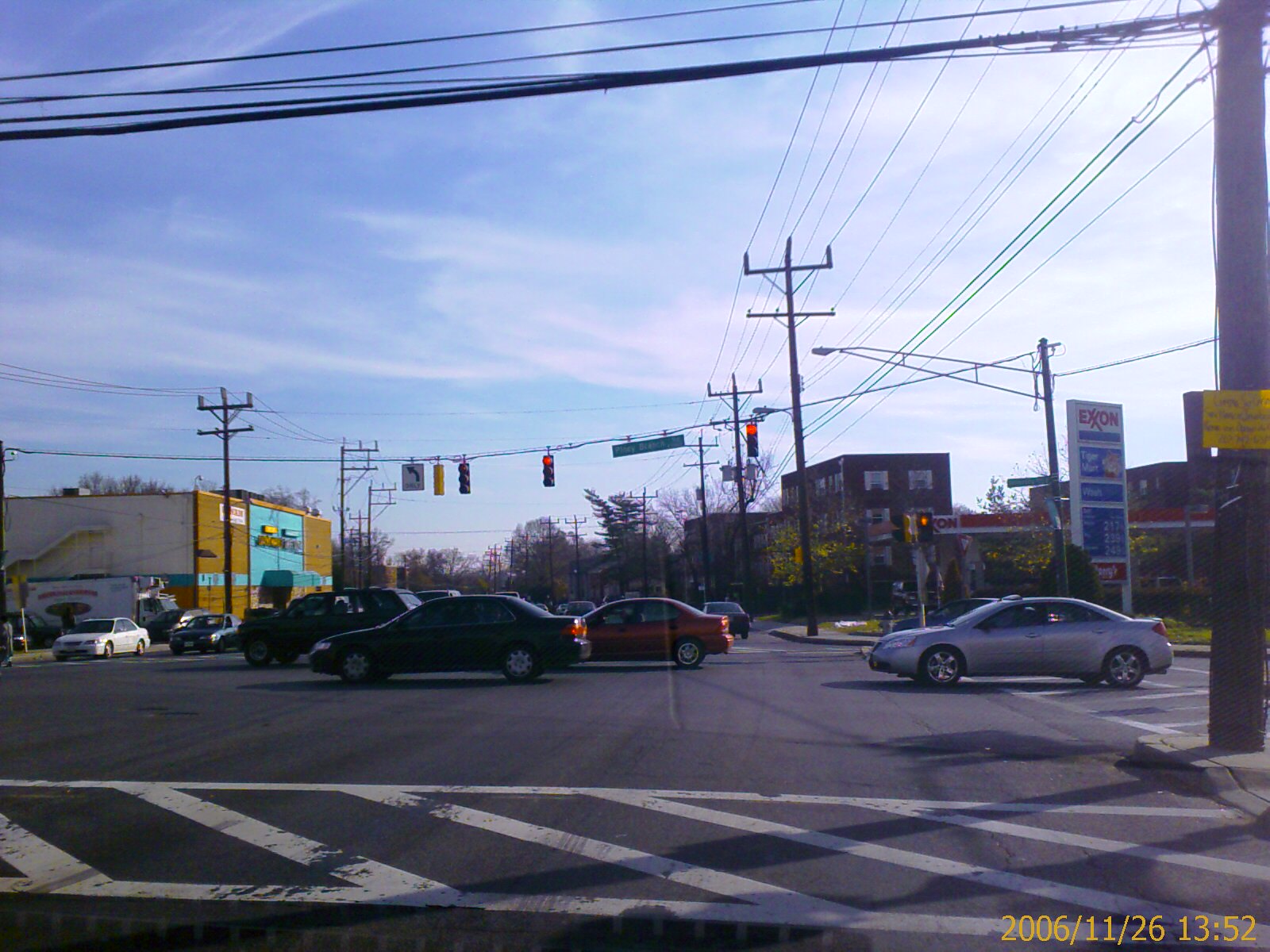The image depicts a bustling intersection with multiple cars navigating through a traffic light system. Situated at the bottom right of the image, a date and time stamp reads "2006/11/26, 13:52." The vantage point appears to be from within a car, possibly through a clean windshield as faint dashboard reflections are visible.

The foreground showcases a white-striped crosswalk on a gray road, leading into a busy intersection. Four cars—a mix of black, red, and silver—are captured moving from left to right under a green light, while additional cars wait at a red light to the left. Distinctive elements include a brown pole with electrical wires stretching horizontally and several lamp and telephone poles dotted across the scene.

On the right-hand side, an Exxon gas station stands prominently, its red-lettered sign displaying gas prices in blue and white patches beneath. Behind the station, brown buildings framed by trees add depth. On the left, another building features a cream white facade with teal blue accents. The overall setting seems to be a commercial or residential area with one to two-story buildings and a network of telephone lines threading through the background.